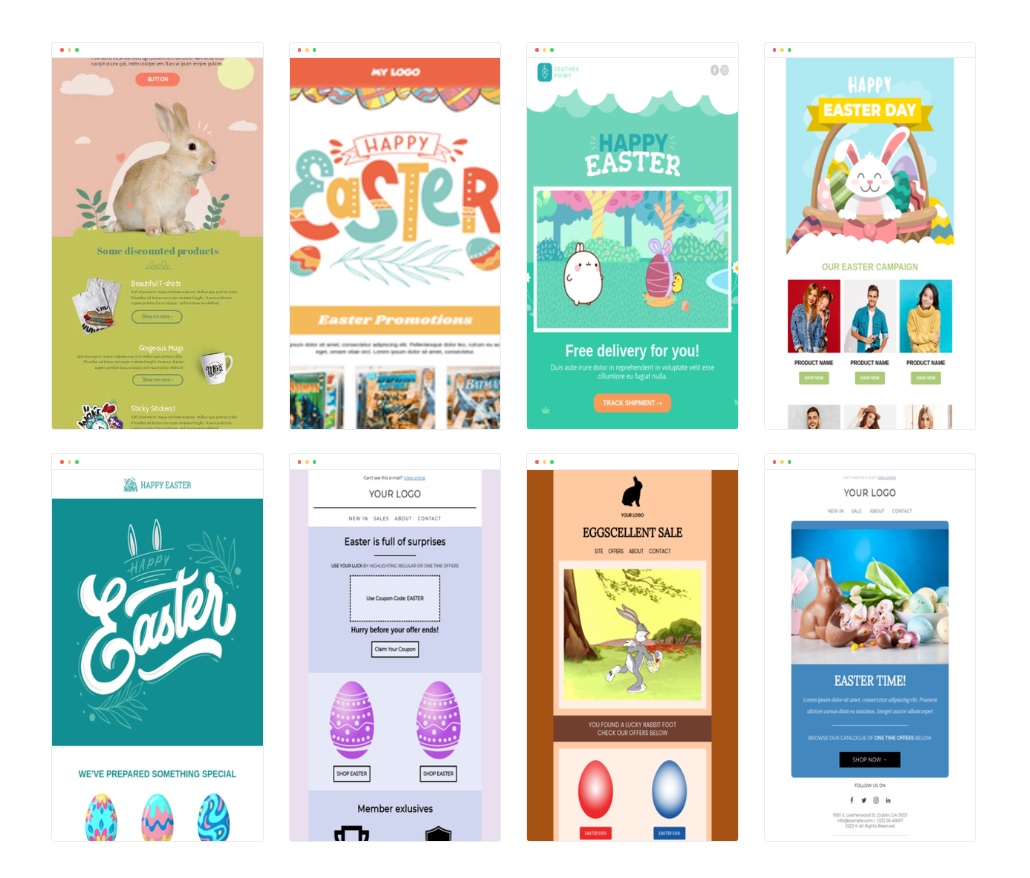A collection of search result thumbnails related to Easter, laid out in a 4x2 grid. The images suggest various ways to personalize Easter-themed cards and gifts, likely for children. 

Top Left: A whimsically designed scene featuring pastel pink clouds and other cutesy elements, possibly for a customizable Easter card.

Bottom Left: A displayed arrangement including a picture frame, a cup, and another item, hinting at personalized Easter gifts.

Top Second from Left: A graphic with the phrase "Happy Easter" and options for customization, suggesting personalized Easter greetings.

Bottom Second from Left: A promotional image offering free delivery on personalized Easter items.

Top Third from Left: Various choices for Easter-themed personalization, potentially for greeting cards or other gifts.

Bottom Third from Left: An advertisement showcasing children’s clothing, suggesting options for Easter outfits.

Top Right: Another customizable Easter-themed option, adding to the array of personalized gift ideas and cards.

Bottom Right: Further promotional content suggesting clothing or other personalized Easter items for children.